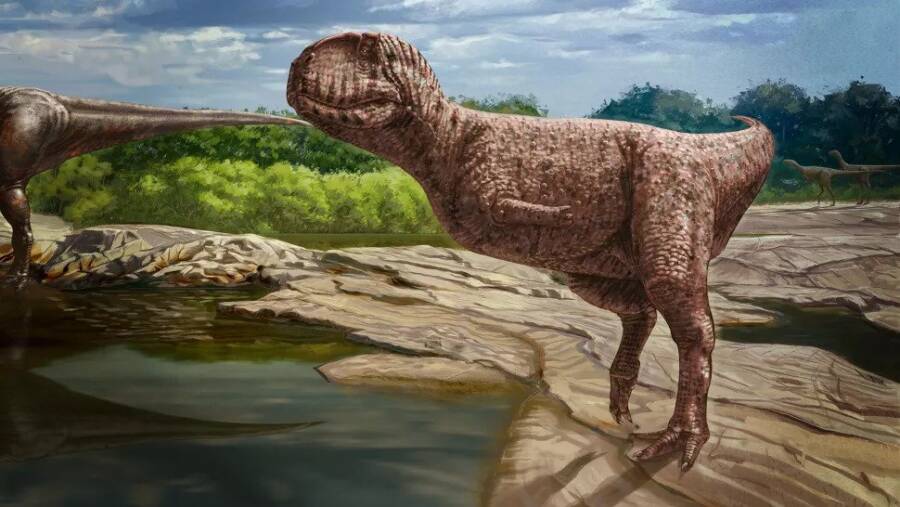The image appears to be a computer-generated or painted scene depicting a detailed profile of a T-Rex-like dinosaur standing on a large granite floor with scattered slate rocks. The dinosaur, characterized by its short arms, long back legs, and wrinkled face, features a brown, spotted, and somewhat aged appearance. Its long tail extends towards another dinosaur's tail and lower body, both reflected in a small body of water among the rocks. The scene is set in a natural environment, with green grass to the left, trees to the right, and a cloudy blue sky above. Additional dinosaurs can be seen in the background, adding depth to the scene.